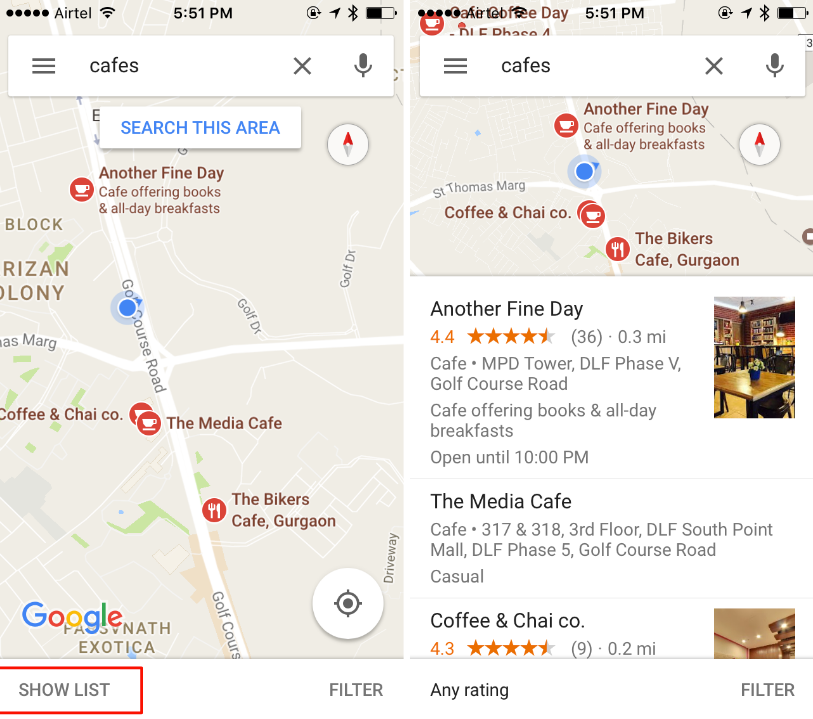This image consists of two side-by-side screenshots of a map interface, such as Google Maps, likely displayed on a mobile device.

**Left Screenshot:**
- The top status bar displays four dots indicating network signal strength, the "Airtel" carrier name, a fully connected Wi-Fi symbol, the time "5:51 PM", and a lock icon within a semi-circle, followed by GPS and Bluetooth icons, and finally, a battery icon showing approximately 50% charge.
- Below the status bar is a white search bar, where the user has typed "cafes" in black text. Beneath the search bar, in white text on a blue background, it says "Search this area."
- The map area displays predominantly gray with white roads. Roads are labeled, with "Golf Course Road" and various similarly named streets such as "Golf Drive."
- The Google logo is positioned in the bottom left corner of the map.
- Also at the bottom left corner, a red square highlights an option labeled "Show list."

**Right Screenshot:**
- The top status bar remains identical to that of the left screenshot.
- In the map section, one of the cafe locations has been selected and more details are visible in a pop-up box.
- The pop-up contains the following information:
  - A search option labeled "Find another cafe" at the top in white text.
  - An orange "4.4" rating followed by four and a half stars and 36 reviews.
  - Descriptive text about the cafe, stating "Cafe Tower" on "Golf Course Road," offering books and all-day breakfast, and indicating it is open until 10 PM. 
  - Additional nearby cafes mentioned include "Metacafe" and "The Coffee and Chai Company."

These detailed captions offer clear insights into the visual elements and functionality presented in the map interface screenshots, highlighting the search for cafes and how the map updates when selecting a specific venue.